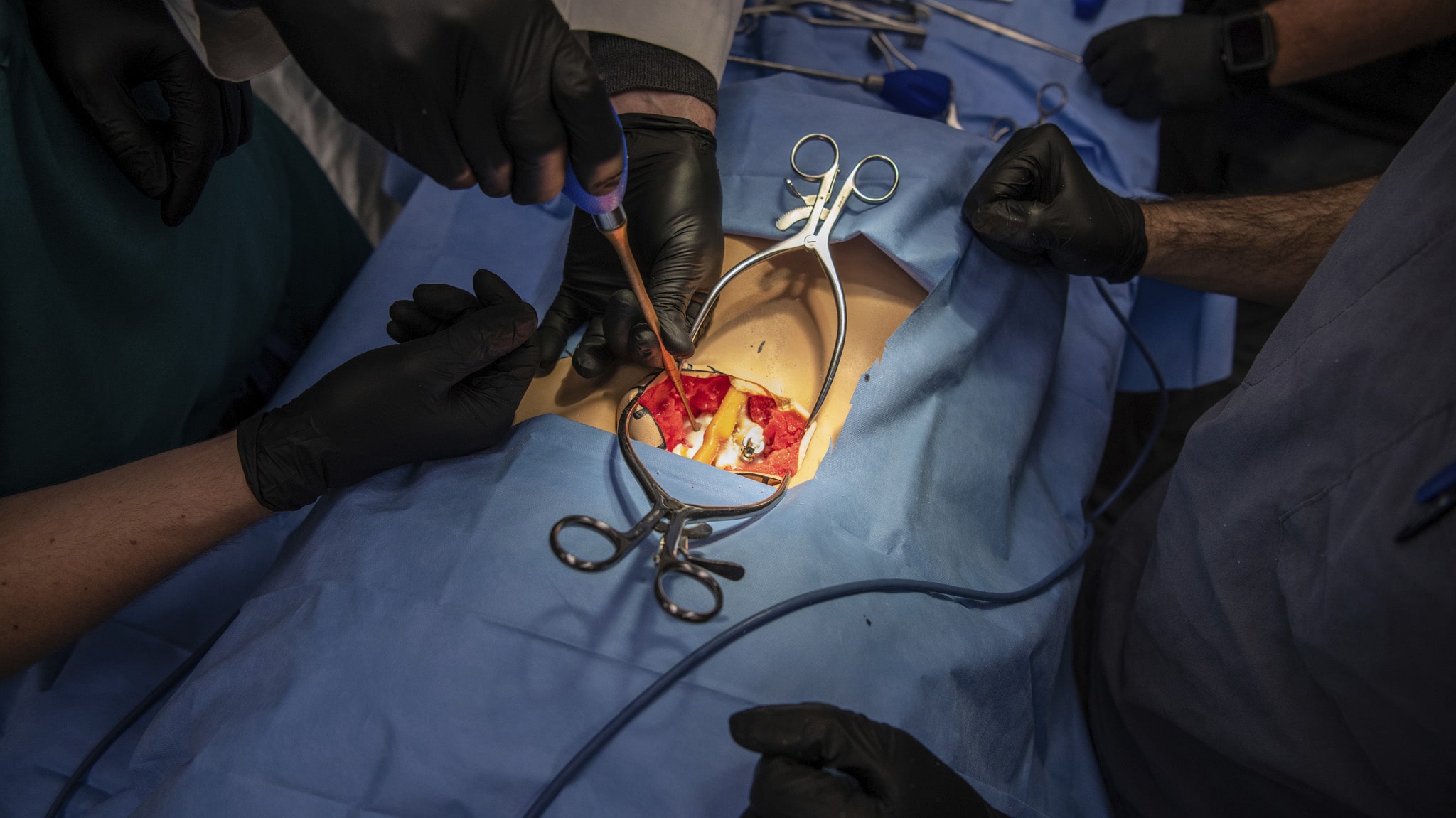The image depicts an indoor surgical setting where a simulated abdominal surgery is being practiced on a 3D printed cadaver. The blue surgical drapes are cut into a square to reveal the pelvic area of the cadaver, showing what appears to be muscles and blood vessels. Large retractors are used to keep the cavity open. On the right side of the operating table, a person, presumably a doctor, is seen wearing a blue scrub shirt and black gloves, although their face is not visible. Another individual on the left, also wearing black gloves, is inserting some type of syringe or instrument into the open cavity. Surgical instruments such as scalpels and suction devices are visible, adding to the realism of the practice environment.